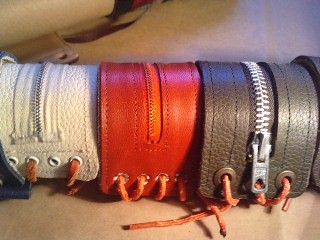The image illustrates three wide, leather wristbands, each fitted with a central zipper running from side to side. The wristbands are arranged in a semi-circular, tunnel-like formation on a wooden table. The colors of the bands from left to right are white, red, and grey. Each wristband features eyelets near the edges, threaded with orange shoelace-like strings, which presumably serve to adjust the fit. The zippers and laces not only add to the aesthetic but also suggest a functional aspect, possibly for securely storing small personal items such as money or credit cards. The overall appearance of these wristbands combines utilitarian and decorative qualities.